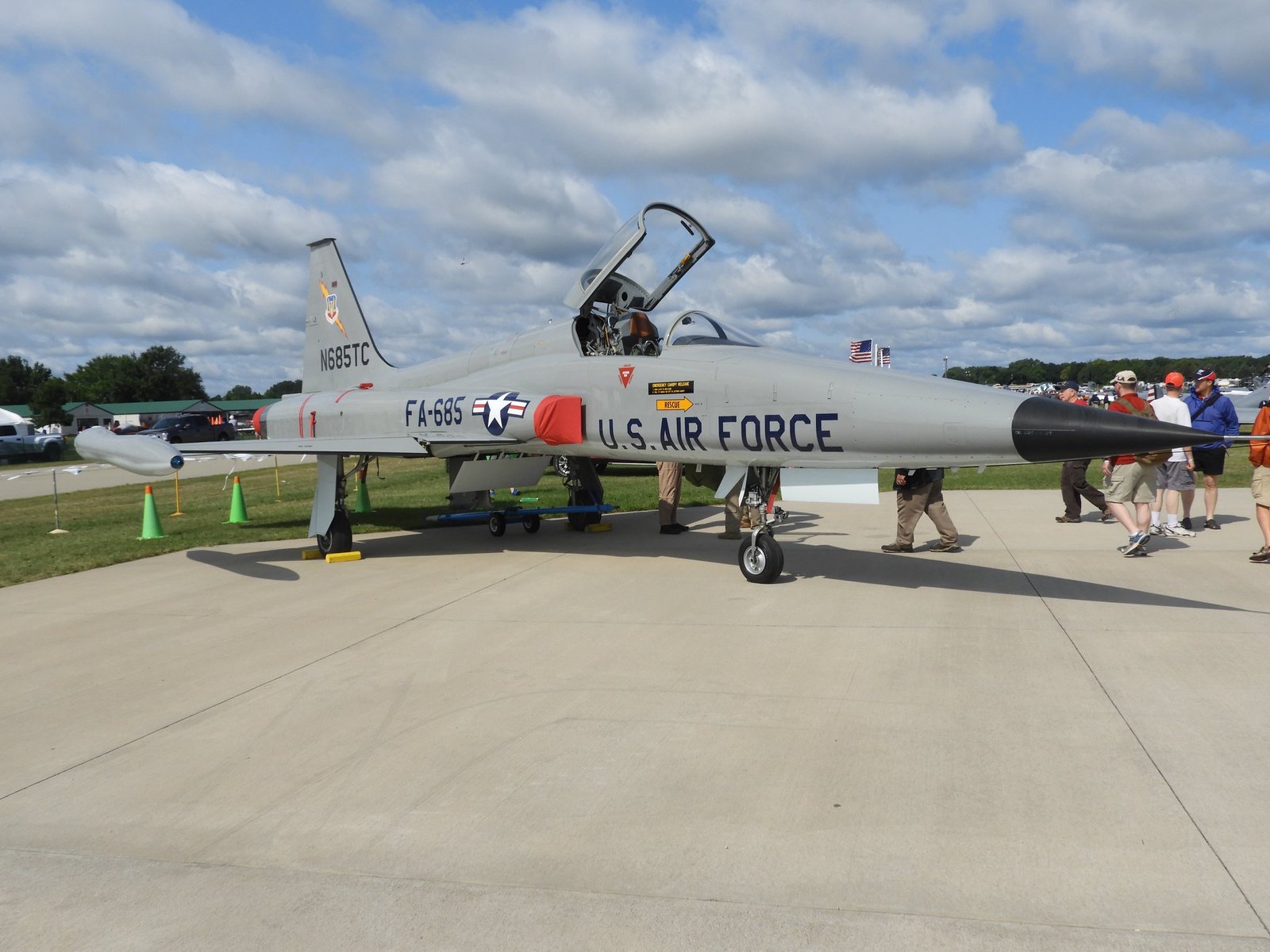This photograph captures a detailed scene at an air show featuring a U.S. Air Force fighter jet, likely an older model, possibly an F-14. The aircraft, primarily a dull gray color, stands prominently on a flat gray concrete surface. It has a black, pointed nose cone equipped with a lightning rod at its tip, and the fuselage displays "U.S. Air Force" in large blue letters beneath the cockpit. A notable feature is the white star inside a blue circle, traversed by a red, white, and blue stripe, located on the rear portion of the fuselage alongside the identifier FA-685.

The background showcases a vibrant blue sky filled with white and gray puffy cumulus clouds. Behind the jet, there's a mix of grass, trees, and what appears to be a taxiway adorned with lime green cones. Various spectators, both to the front and back of the aircraft, are visible, admiring the jet. The cockpit is open for public viewing, further indicating the air show setting. Another marking, N685TC, is seen on the tail wing, along with a logo emblazoned on the tail fin, adding to the jet's distinct appearance. This setting, combined with the jet's sleek and pointed design, makes for a compelling and dynamic scene.